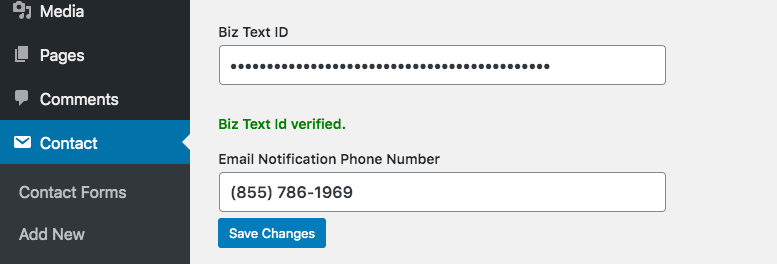The image portrays a rectangular interface layout, with its left quarter shaded in black. This black section functions as a sidebar, containing six vertically stacked clickable items. Each item is represented by an icon and a label. From top to bottom, the items are as follows:

1. **Media**: Accompanied by a camera and music notes icon.
2. **Pages**: Represented by a sheet of paper icon.
3. **Comments**: Indicated by a speech bubble icon.
4. **Contact**: Currently highlighted with a white font and an envelope icon. The entire highlighted section, including the envelope icon, is white, while the rest of the items are in blue. A small arrow on the right side of this item indicates it's currently selected.
5. **Contact Forms**: Displayed in a gray font.
6. **Add New**: Suggestively indicating an option to create something new.

On the right side of the interface, details related to the highlighted "Contact" section are displayed. It includes:

- **Biz Text ID**: A long dotted entry field, likely intended to conceal a code or password, spanning approximately 20 characters.
- **Biz Text ID Verified**: A confirmation label.
- **Email Notification**: Presumably, a field or setting related to email alerts.
- **Phone Number**: A visible phone number is displayed here, which is notably unusual.
- **Save Changes**: A blue button available for saving any modifications made.

The detailed layout highlights navigation options on the left with corresponding functionalities on the right, geared towards managing contact details.